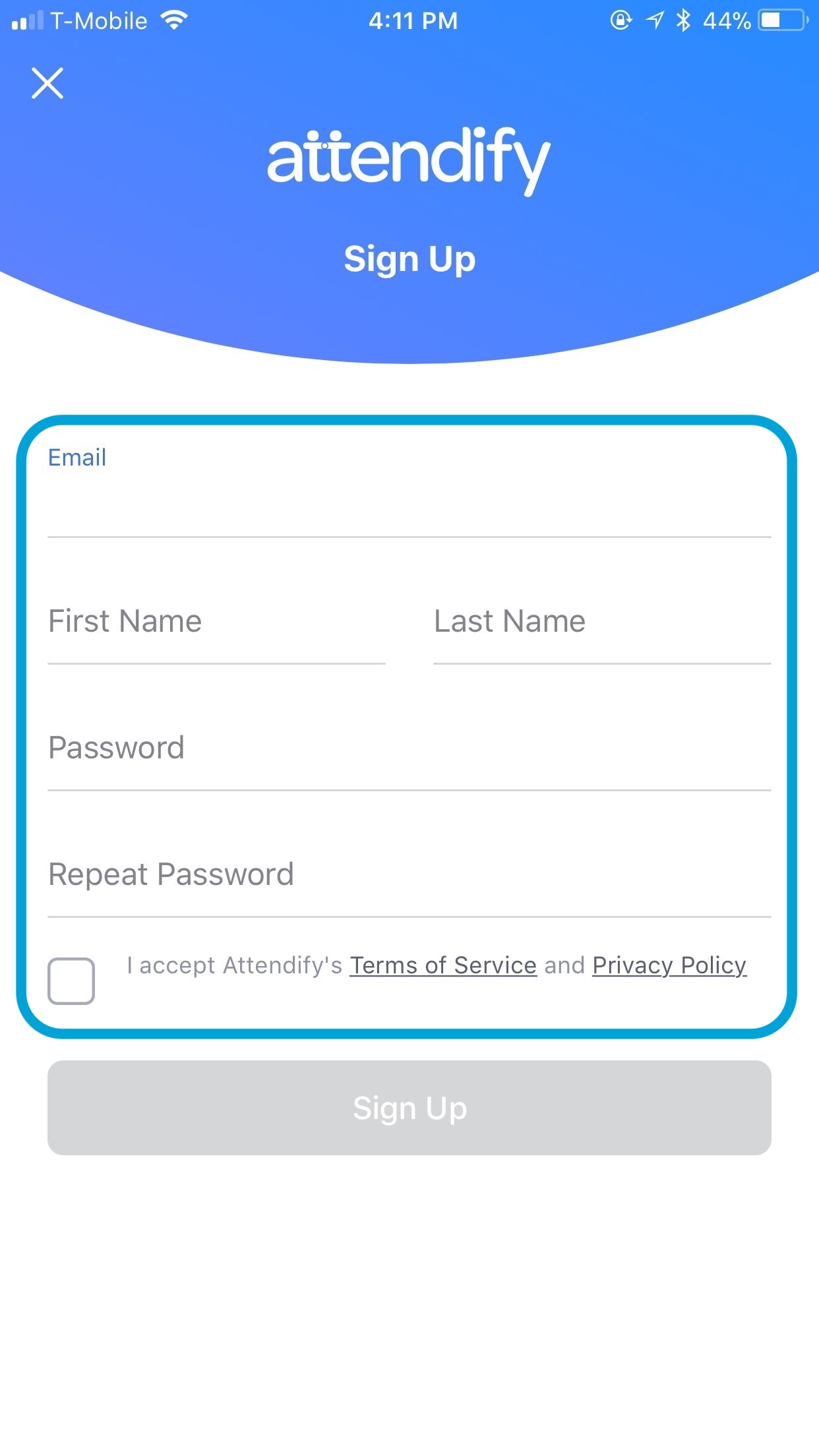This image is a detailed screenshot from a T-Mobile cell phone captured in portrait orientation. The background is predominantly white, providing a clean and minimalistic look. At the top of the screen, there's a medium-blue banner with a curved bottom edge. Within this banner, white text is displayed. 

In the top-left corner, the T-Mobile carrier information is visible along with two cellular signal bars. Centrally positioned at the top, a Wi-Fi signal icon is shown. Next to it, the time is displayed as "4:11 p.m." On the top-right, there are icons for Bluetooth connectivity and a battery indicator at 44%.

Beneath this banner, aligned flush left, there is an "X" symbol. Below it, in larger white text, is the word "Attendify," with distinctive dots placed above the crossbars of both "T's." Further down, in smaller white letters, the option to "Sign up" is provided.

Following the curved bottom edge of the blue banner, the screen transitions to white. Below this, there is a rectangular input form outlined in teal blue with rounded corners. This form includes fields to enter "Email," "First Name," "Password," and "Repeat Password." Below these fields, there's a checkbox option on the bottom left, where users can agree to Attendify's terms of service and privacy policy by selecting "I accept Attendify's terms of service and privacy policy."

Finally, at the very bottom of the screen, there's a grayed-out bar centrally displaying the text "Sign up" in white print, indicating the button for finalizing the registration process.